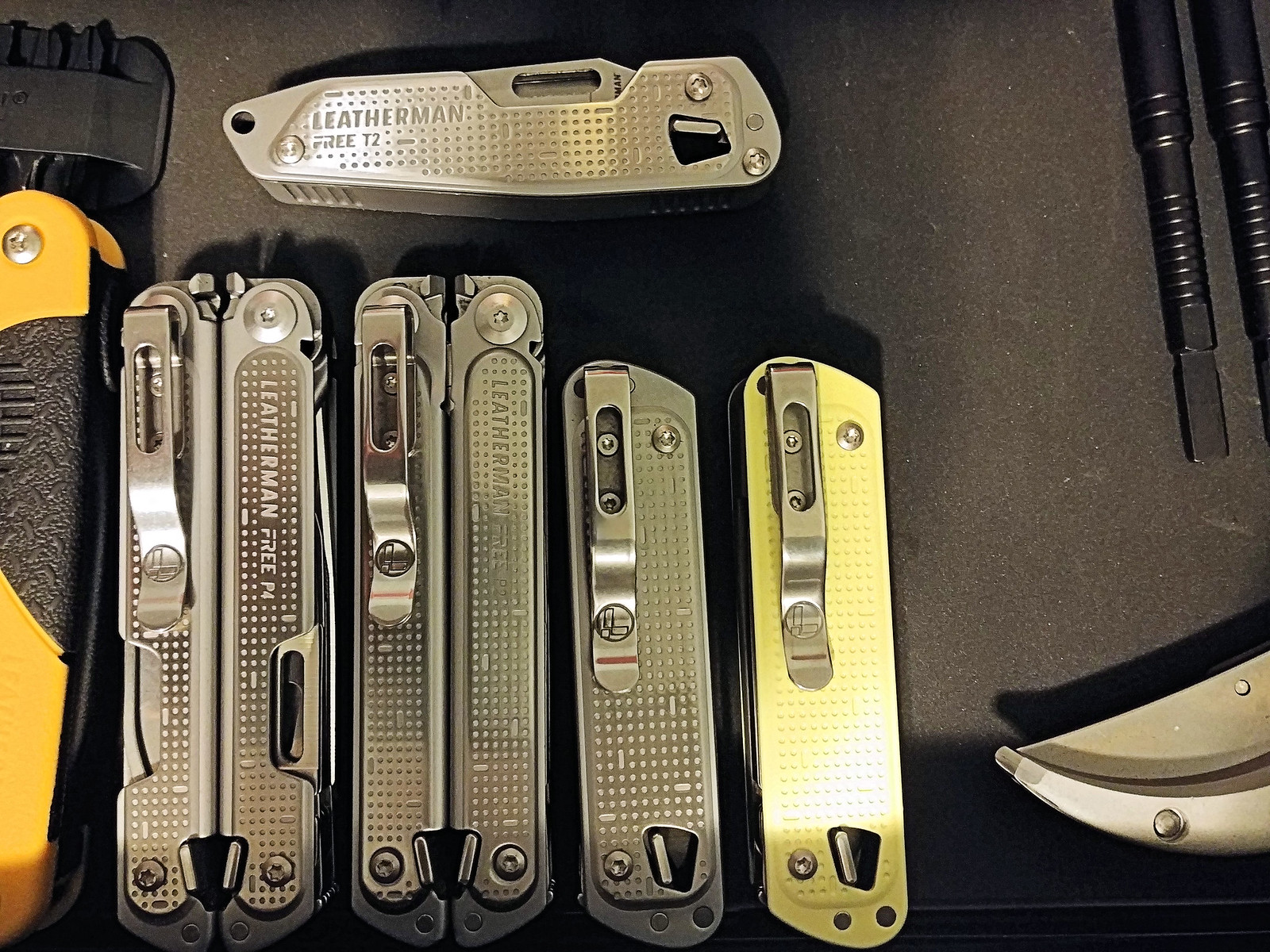On a dark grey to black table surface lies an array of multi-tools and utility knives, predominantly branded as Leatherman. Central to the scene, there are five fully visible multi-tools: four are silver-colored, and one on the far right has a yellowish or golden hue with a silver clip. To the left, a partly visible multi-tool features a yellow and black design. One multi-tool, slightly apart and positioned on the right side, is primarily yellow. Overlapping descriptions emphasize the distinct presence of black tubular metal pieces in the top-right corner, which appear to be screwdriver heads or drill bits. There is also mention of another cutting tool that resembles pruning shears. Additionally, three of the multi-tools are marked as "Leatherman Free" models, denoting different variants like P4, P2, and T2. The meticulous arrangement and diversity of the tools suggest preparedness and utility, capturing the essence of a robust toolkit on display.